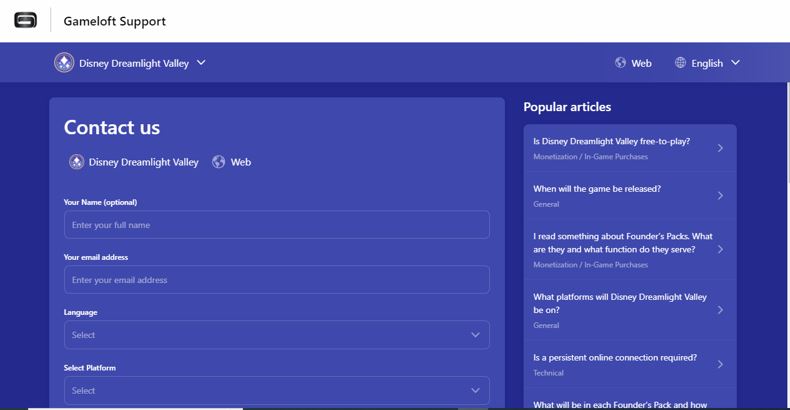The web page features a clean and organized layout with a prominent dark blue color scheme. At the top of the page, a light-to-dark blue gradient rectangle spans across the header, providing an eye-catching contrast. Positioned in the top left corner, there is a gray circle adorned with white diamond shapes. To the right of this circle, the text "Disney Dreamlight Valley" is displayed, accompanied by a downward arrow indicating a dropdown menu.

On the top right corner, there are icons including a globe labeled "web" and another globe labeled "English," also accompanied by a downward arrow for language selection.

The main content is divided into two sections. The left side, slightly extending past the middle of the page, contains a form with a lighter blue border. This section is labeled "Contact Us - Disney Dreamlight Valley Web." Inside this area, there are input fields for users to enter their name, email address, select their language, and choose their platform.

To the right, there is a smaller box titled "Popular Articles." This section lists several FAQs with right-pointing arrows for further navigation. The articles include:
- "Is Disney Dreamlight Valley free to play?"
- "When will the game be released?"
- "I read something about Founders Packs, what are they and what function do they serve?"
- "What platform will Disney Dreamlight Valley be on?"
- "Is a persistent online connection required?"